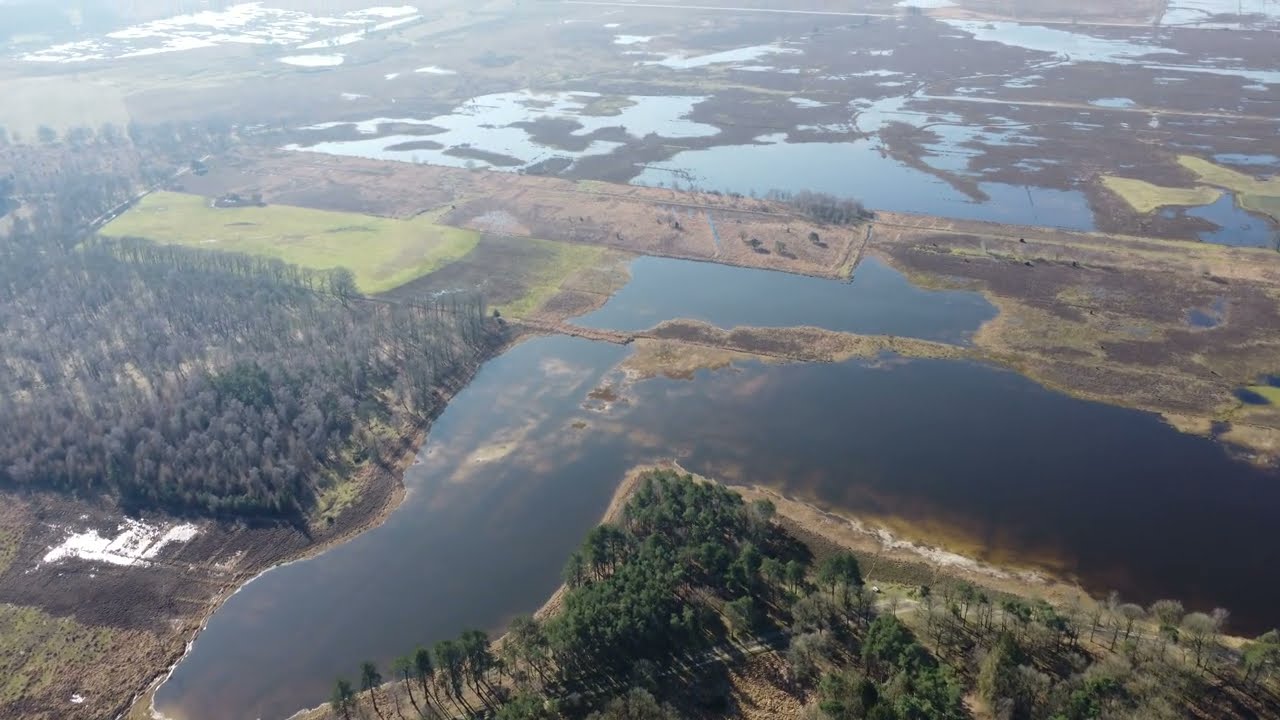This aerial color photograph, captured from a considerable altitude—perhaps using a drone, plane, or helicopter—depicts a vast, marshy landscape. Dominated by large and small patches of water that appear to intersperse the terrain, the scene resembles a floodplain or swampy area where water has overtaken much of the land. To the left and bottom of the image, dense clusters of trees, including leafless tall trees and pine trees, frame the watery expanse. In the foreground, a footbridge extends halfway across the water towards the opposite bank, suggesting intermittent human presence. The overall impression is that of a wetland area, possibly the result of recent flooding, with few visible roads and a mixture of sprawling forest and grassy fields. The absence of urban features emphasizes the natural, untamed quality of the landscape.